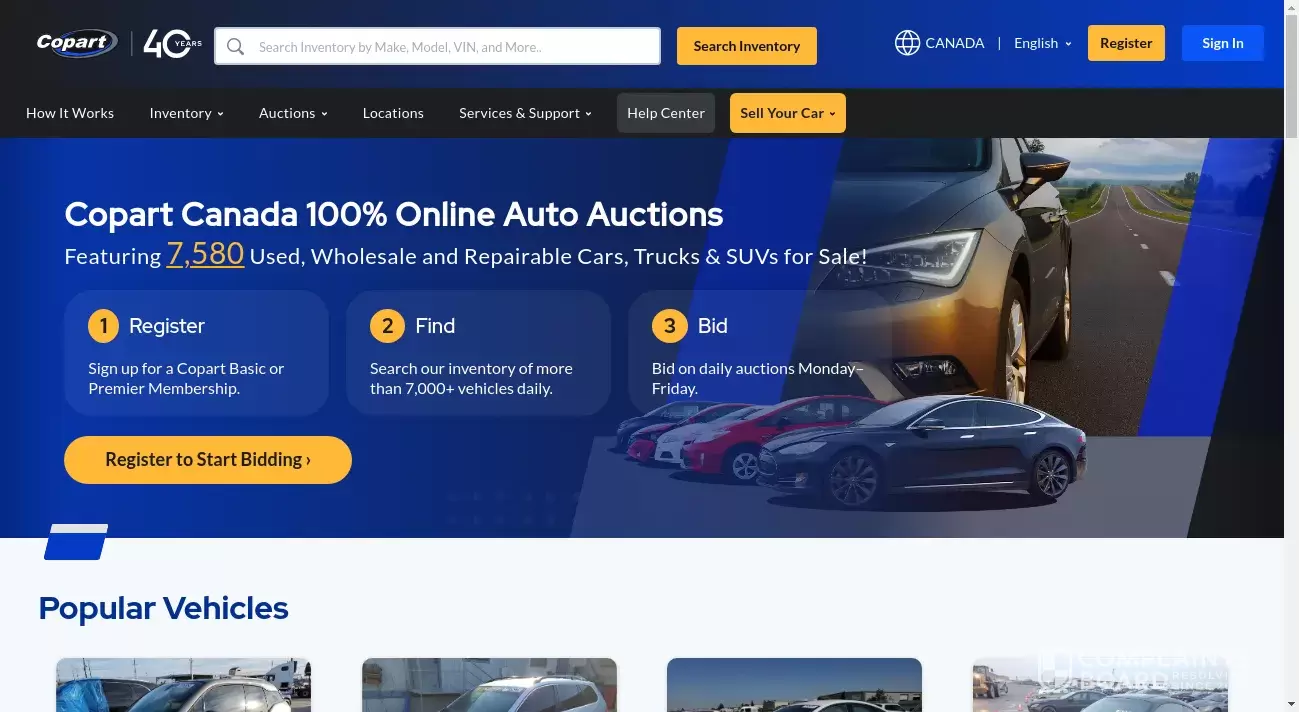The image is a screenshot of the homepage of Copart, an auto auction website celebrating its 40th anniversary, as indicated by the "40 years" logo where the zero incorporates the word "years." To the right of the logo, a search bar is prominently featured, allowing users to search the inventory by make, model, VIN, and more. Adjacent to the search bar is a yellow button with blue or black text that reads "Search Inventory."

Further right, a global icon with the word "Canada" is displayed, suggesting the geographic location. Next to this is a language selector, with English currently chosen. Following this, a yellow "Register" button with black text invites new users to sign up. Beside it, a blue button with white text provides the option to "Sign In."

Below these primary features are a series of navigation menus: "How It Works," "Inventory," and "Auctions" (indicated by a small down arrow for additional options). Further to the right are "Locations," followed by "Service and Support," which also suggests additional options with a down arrow. Near the far right is a dark gray "Help Center" button with white text, and finally, a yellow "Sell Your Car" button with dark or black text for users looking to sell their vehicles.